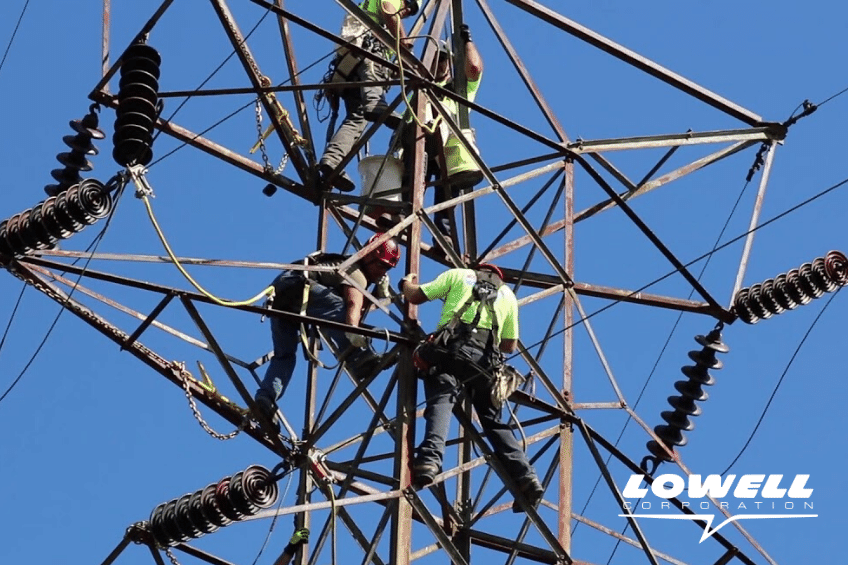This detailed color photograph, oriented in landscape mode, captures a high-angle view of four workers stationed on an expansive electrical substation tower. The central metal structure of the tower rises with interconnecting fretwork, extending laterally towards the left and right at the top. Looming large against a backdrop of clear blue sky, the photograph highlights the formidable height and intricate design of the electrical post, adorned with black circular rings to hold the overhead wires.

The men, equipped with helmets and climbing gear, are stationed at different levels of the tower. Two workers are visible at the top, facing each other, while the two others are positioned lower below the center section, also engrossed in their tasks. Most of the men are dressed in bright yellow or green shirts with red hard helmets, though one worker is distinguishable by his orange hard hat, black trousers, and tool belt around his waist. The scene of their collaborative effort is underscored by the presence of multiple transistors and extensive wiring, emphasizing the complexity of the electrical structure they are working on.

In the lower right-hand corner of the photograph, 'Lowell' is prominently printed in white, with 'Corporation' beneath it, underlined with a heartbeat line, affirming the image's association with the company.